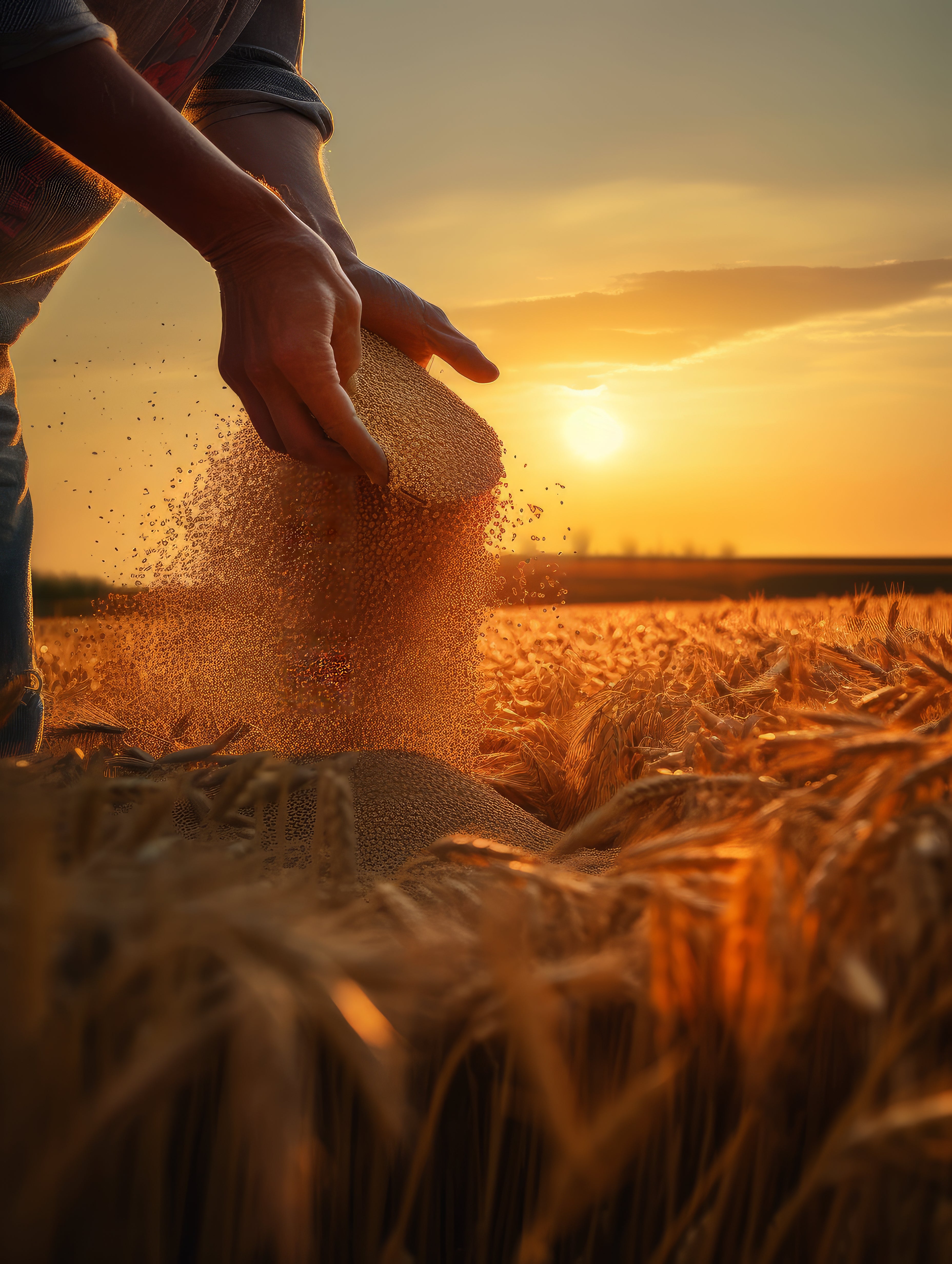In this image, a pair of human hands with medium-toned light skin is prominently featured. The hands are gender-neutral, not indicating a specific gender. The sleeves of a shirt are rolled up to just below the elbows, and a sliver of gray pants is visible at the bottom of the frame. The hands are cupped around an aggregate or grain, which appears to be pouring from an obscured, rectangular container with rounded edges. This grain is falling into a pile on the ground, surrounded by a field of tall, yellow grass or wheat. In the background, a vibrant yellow sun is positioned low on the horizon, suggesting either sunrise or sunset. The sky transitions from a rich yellow near the horizon to light blue at the top, with scattered clouds reflecting the golden hue.